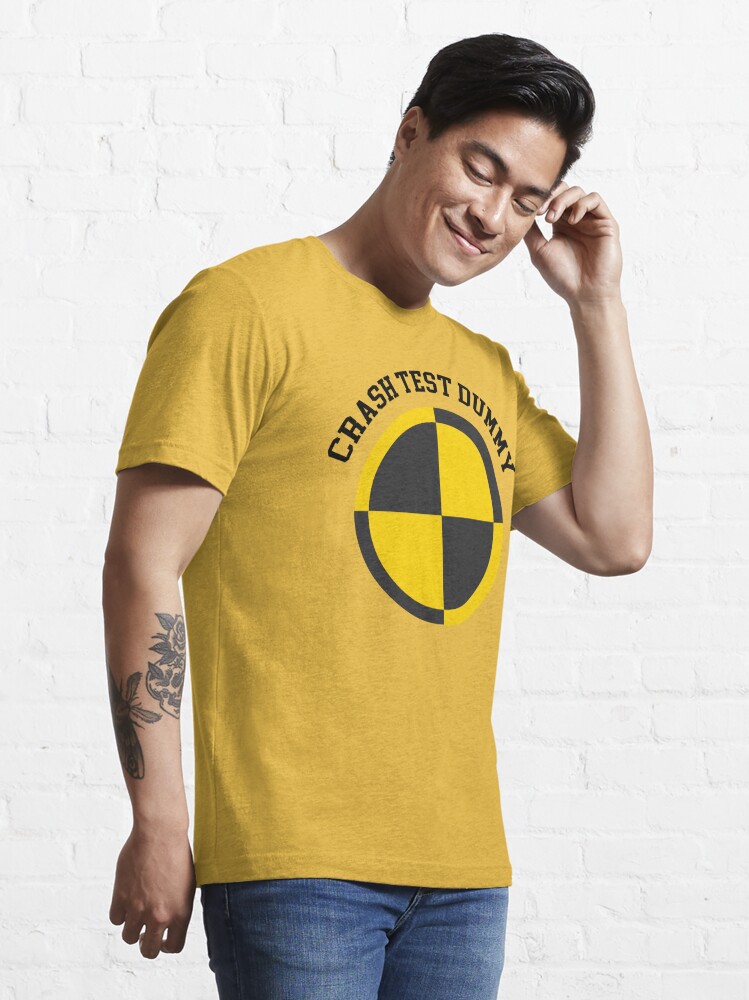A vertically oriented color photograph showcases a man posed against a white brick wall, resembling an advertisement for a t-shirt. The man, with dark hair combed to the sides and a slight smile, stands with his left hand up to his left ear, tilting his head slightly downward. He's wearing a maize or dark yellow t-shirt prominently featuring a crash test dummy design in the center. The design consists of a circle with four yellow and black quadrants, with the words "Crash Test Dummy" arched above it. His outfit is completed with blue jeans. His right arm, resting by his side, reveals a detailed tattoo extending from the inside of his elbow to the forearm, including a skull with a rose and possibly a butterfly. The t-shirt appears to be a blended fabric, giving it a textured look with various darker shades interwoven into the yellow. The overall setting and his slightly closed eyes suggest a relaxed and cheerful vibe.